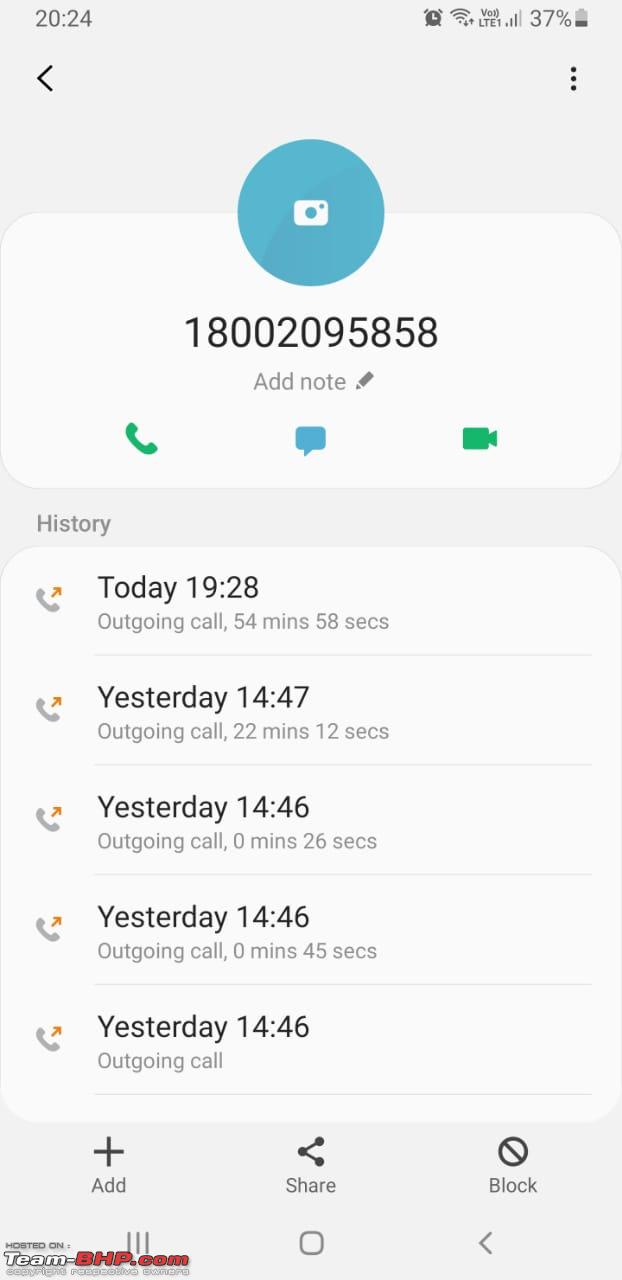This screenshot captures a detailed view of the call history screen of a cell phone for a specific contact. In the top left corner, there's a label indicating this section is for the history of calls with a contact, and the current year, 2024, is displayed in the top right. The status bar at the top shows icons for an alarm clock, Wi-Fi signal, cell service, and battery, which is at 37%.

Moving down, the contact information is displayed prominently. The phone number, 1-800-209-5858, is highlighted beneath a placeholder image—a blue circle with a camera icon, indicating no photo is assigned to the contact. Next to the phone number is an option to 'Add note,' illustrated with a small pen icon.

Just below this are icons for making a phone call, sending a text message, and initiating a video call. The call history is listed below these options, starting with today’s entry at 19:28 for an outgoing call that lasted 54 minutes and 58 seconds.

Yesterday's entries are detailed thereafter:
- At 14:47, an outgoing call lasting 22 minutes and 12 seconds.
- At 14:46, another outgoing call lasting 26 seconds.
- Another outgoing call at 14:46 lasting 45 seconds.
- A final entry at 14:46 indicates an outgoing call with no duration shown.

At the bottom of the screen are options to add the contact, share it, or block it, denoted by a plus sign, a share symbol, and a circle with a cross through it, respectively. The bottom navigation bar includes icons for home, back, and menu, helping users navigate the application's interface.